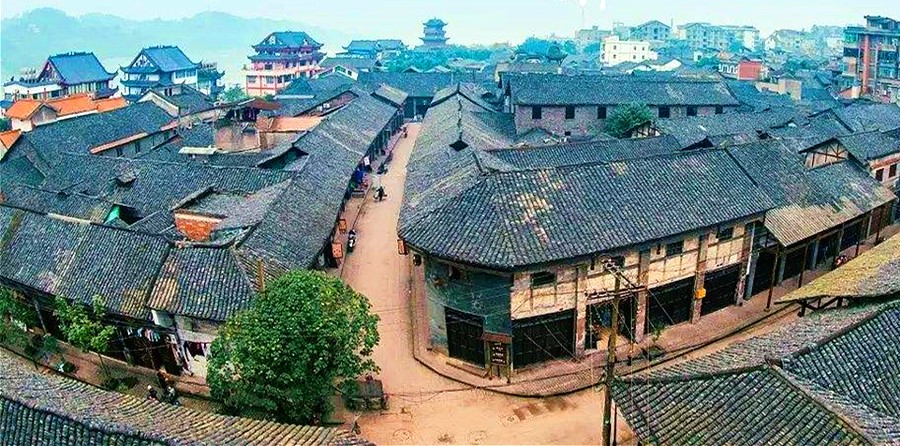This image is a colorful, wide-angle photograph of a city street in an Asian city, potentially Japanese or Chinese, captured during the daytime. The wide-angle lens distorts the scene slightly, giving everything a curved appearance. The foreground features a dark brown, muddy street lined with parked motorcycles or mopeds. Several buildings with gray and black gabled roofs show signs of wear and tear, with visible patches and areas undergoing repair, marked by exposed plywood and bricks. The architecture of these buildings reflects traditional Asian styles, characterized by their curved, upward-tilting tips and temple-like designs.

To the left, green-leaved trees line the street, providing a touch of nature amidst the urban setting. Multi-story buildings with newer construction and more modern appearances are evident in the background on the right. Also prominent in the background are mountains, adding a natural contrast to the cityscape and enhancing the depth of the scene.

At the center of the furthest background stands a tall, traditional pagoda tower, embodying the cultural essence of the city. Surrounding it, especially to the right, are various multi-story constructions that look fresher and less worn. Despite the traditional appearances of many structures, modern elements such as power lines can also be seen, blending the ancient with the contemporary. The overall scene captures a vibrant juxtaposition of old and new, within a distinctly Asian architectural setting. No text is present in the image, allowing the visual narrative to speak entirely for itself.